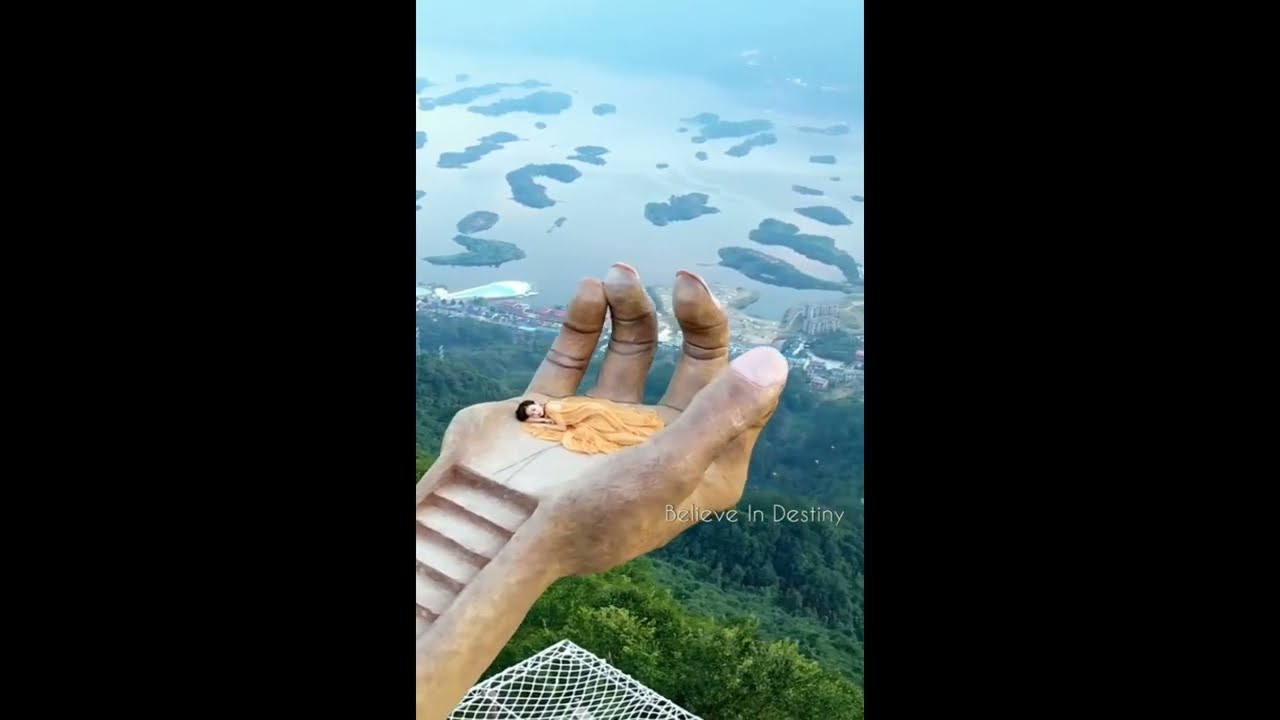The image portrays a striking hand statue with fingers bent upward, forming a grand staircase along the wrist. At the top, in the open palm, a woman lies draped in a flowing yellow dress, as if asleep, creating a serene focal point. Below this monumental sculpture, lush green trees blanket the landscape, stretching down a verdant mountain or large hill. Beyond this rich greenery lies a vast, blue ocean dotted with small islands and flanked by a bustling coastline, featuring buildings meticulously arranged along the shore. The overall scene is tinged with colors of dark and light green, light orange, brown, white, and black. Adding a touch of inspiration, the image includes white text towards the lower right, reading "Believe in Destiny." The photograph, taken from an elevated angle during the daytime, captures an enchanting fusion of nature and art, emphasizing the grandeur and contemplative serenity of the statue and its surroundings.